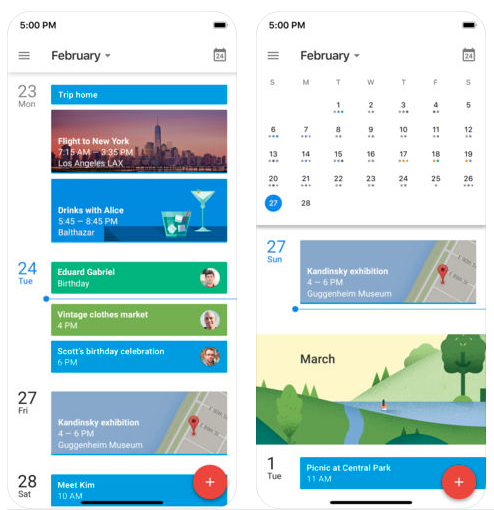*Dual Screenshot of a Busy Scheduler on an iOS Device*

In this side-by-side pair of screenshots, we see a detailed view of an iOS calendar app, identifiable by the bottom navigation bar used to exit the app. Both screenshots display the time as 5 PM with a fully charged battery, and a hamburger icon that offers further options. 

**Date and Day Details:**
- The date header shows "February 24th" alongside a dropdown menu for changing the date.
- Below, it states "23rd Monday," indicating the start of the week.

**Monday, February 23rd:**
- **Trip Home:** Highlighted in a blue rectangle, this event shows a picture of New York with details: "Flight to New York 7.15 AM to 3.35 PM from Los Angeles (LAX)."
- **Drinks with Alice:** Below this, a cartoon image of two alcoholic drinks on a pale blue background states: "Drinks with Alice 5.45 PM to 8.45 PM at Balthazar."

**Tuesday, February 24th:**
- **Edward Gabriel's Birthday:** Marked in medium green, this event features a picture (presumably of Edward Gabriel) and indicates "Edward Gabriel's Birthday."
- **Vintage Clothes Market:** In a paler, olive green, it mentions: "Vintage Clothes Market at 4 PM," accompanied by a generic image of a head.
- **Scott's Birthday Celebration:** Highlighted in blue, showing another man's picture, it reads: "Scott's Birthday Celebration at 6 PM."

**Friday, February 27th:**
- **Kandinsky Exhibition:** Featuring a map pin icon, it notes: "Kandinsky 4-6 PM at the Guggenheim Museum."

**Saturday, February 28th:**
- In medium blue text on a white background, it states: "Meet Kim at 10 AM."

**Overall Calendar View:**
- A comprehensive calendar of February is shown with various colored dots below each date, likely representing different events.

**Sunday, February 27th:**
- Repetition of the Kandinsky exhibition details noted earlier.

**March Events Preview:**
- An outdoor scene presumably depicting a park introduces: "Tuesday the 1st," with a blue rectangle and white text indicating: "Picnic at Central Park 11 AM."

The series of events lined up demonstrates a particularly busy schedule for the user, showcasing a mixture of personal celebrations, social gatherings, and cultural events.